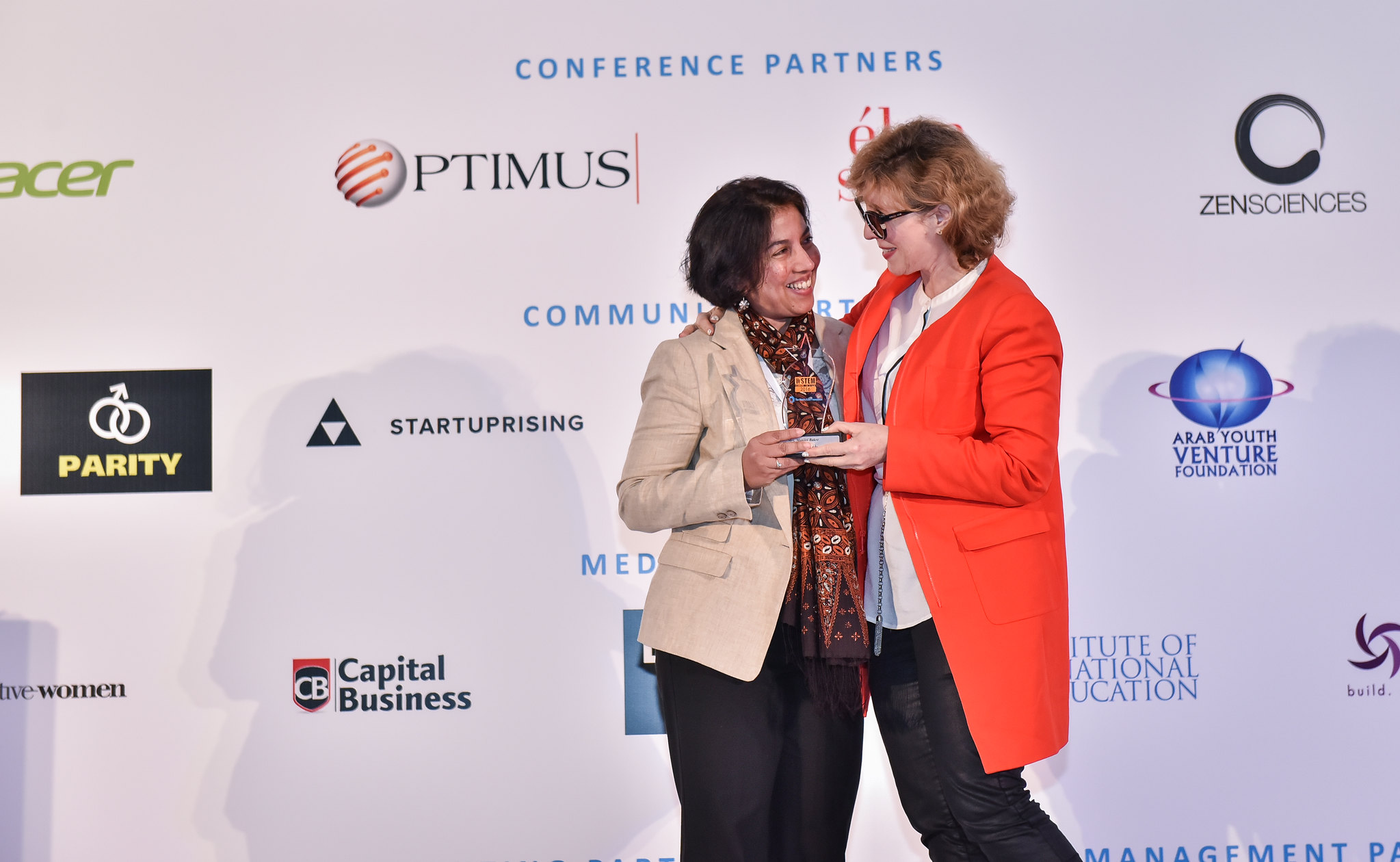In the center of this indoor conference photograph, two well-dressed women are embracing and smiling at each other. The woman on the left, with short dark hair, is dressed in a light tan blazer, dark pants, and a multicolored scarf. She has her right hand extended, appearing to receive a clear-backed award from the woman on the right. The woman on the right has short brown hair and glasses, wearing an orange blazer over a white shirt and dark pants. The background features a large board covered in various sponsor logos and advertisements, including names like Zen Sciences, Arab Youth Venture Foundation, Capital Business, Start Uprising Parity, and Acer, under a heading that reads "Conference Partners." The sponsorship backdrop is vividly colorful with hues of white, green, black, yellow, red, orange, tan, brown, blue, and light blue. The image is cut off below the women's knees, making them slightly right of center as they engage warmly with each other.